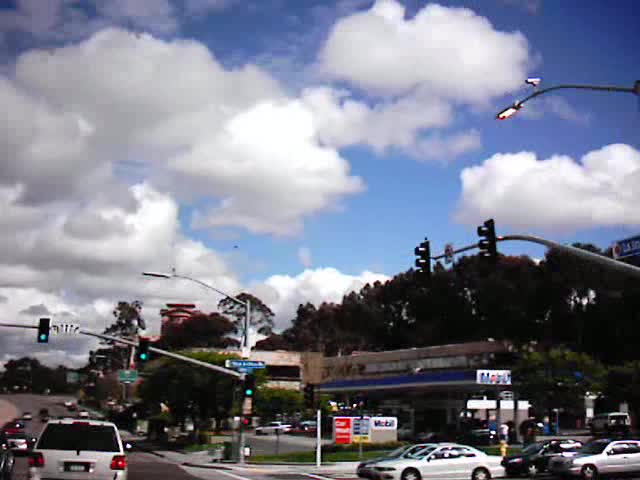A vivid street scene at a bustling city intersection. The foreground features a busy road with multiple cars navigating through the traffic lights, while others await their turn at a cross street on the left. Overhead, the sky is a brilliant blue, adorned with puffy white clouds that highlight the clear weather. A row of tall, mature green trees lines the background, providing a lush contrast to the urban setting. Prominently displayed behind the trees is a long gas station, easily identifiable by its extensive blue awning and the "Mobil" sign. Streetlamps are strategically placed around the intersection, one of which is equipped with a traffic camera, ensuring safety and monitoring. This dynamic photograph captures the essence of city life, blending natural and man-made elements seamlessly.